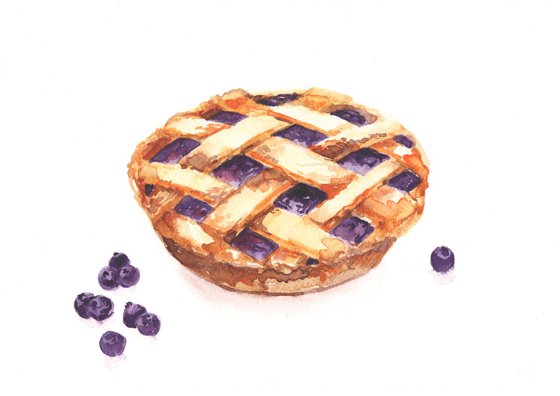The image features a highly detailed drawing of a baked blueberry pie set against a stark white background. The pie itself has a beautifully rendered lattice crust, showcasing a range of tan, light brown, and dark brown hues indicative of a freshly baked golden crust. The lattice pattern exposes the rich, glossy, purple-blue filling, suggestive of a succulent blueberry interior. The artistic detail includes highlights and shading that give the blueberries a jellied, shiny appearance, enhancing their realism. Scattered around the pie on the white background are several individual blueberries: about eight to the left of the pie and one to the right. The careful arrangement and intricate color work make this drawing strikingly lifelike, reminiscent of a traditional grocery store pie advertisement.